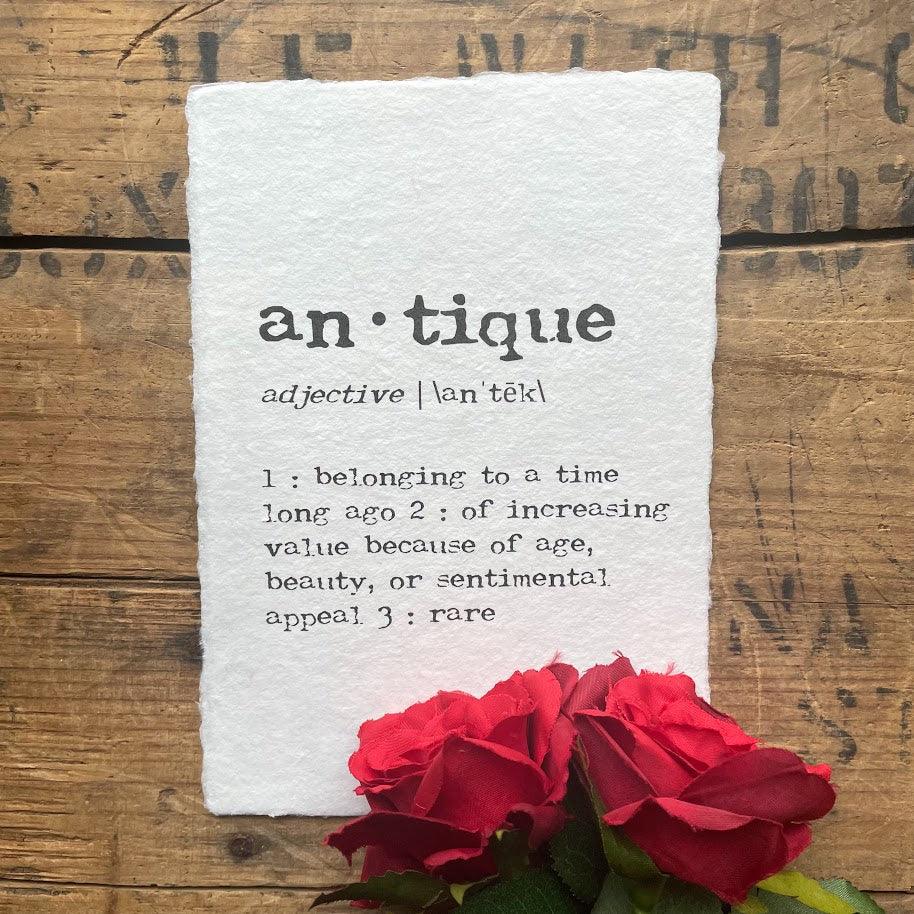The photograph captures a scene with a rustic and vintage essence. In the foreground, the tops of two roses, with their petals slightly fringed, form a triangle as they angle towards the upper corners of the image. Behind them, a piece of textured, handmade paper appears pinned or laid against a backdrop of rough-hewn wooden boards, resembling an old shipping crate with barely discernible, weathered stamped letters and numbers. The paper presents a dictionary-style entry for the word "antique," broken into syllables "an-dot-teak" and identified as an adjective. The definition reads: "1. Belonging to a time long ago. 2. Of increasing value because of age, beauty, or sentimental appeal. 3. Rare." The contrast of the delicately aged text against the coarse wooden background and the artificial roses captures a sense of nostalgia and timelessness.